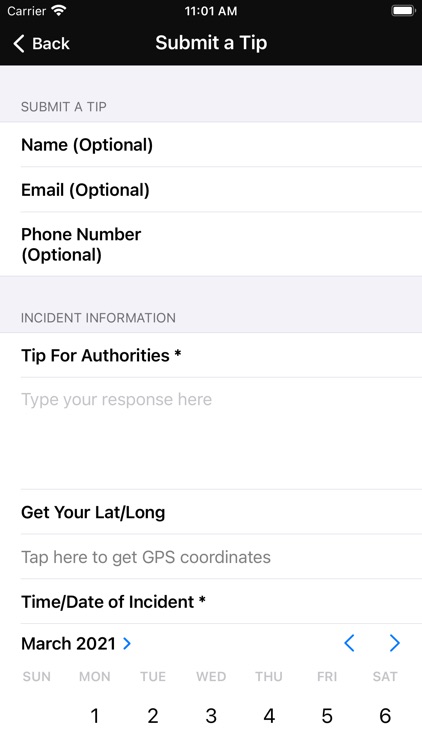The image displayed on the phone screen showcases a user interface of an app designed for submitting tips to authorities. The top section of the screen indicates the current time as 11:01 a.m. The form includes several fields, most of which are optional. Users can enter the name of the tipster, their email address, and phone number. Below that, there is a section labeled "Incident Information," prompting the user to provide detailed information for authorities. A text box is available for the user to type their response.

Further down, there is an option to retrieve the device's GPS coordinates by tapping a specific button. The form also requires users to input the date and time of the incident, with a currently open field displaying March 2021, adjustable via adjacent arrow icons. The app seems to be structured systematically, guiding users to fill the requested information sequentially. This interface appears to be designed for reporting actionable advice or information to authorities, rather than giving financial tips.